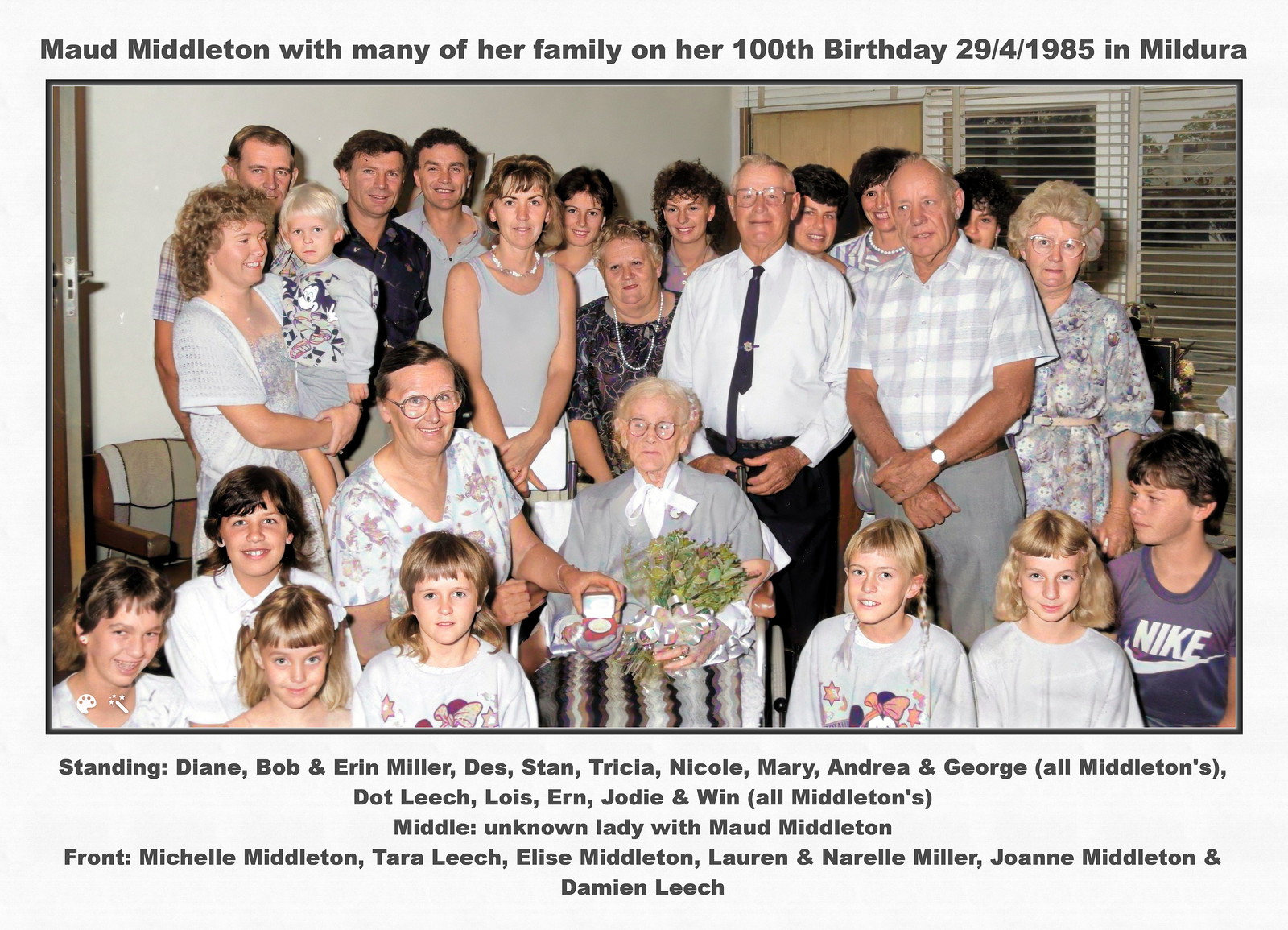The photograph depicts a large extended family celebrating Maude Middleton's 100th birthday on April 29, 1985, in Mildura. The image is crisp and clear, a telltale sign of the 1980s, as evident by the hairstyles. A white room serves as the backdrop, with a window on the right that almost offers a glimpse of distant mountains. At the heart of the photograph sits Maude Middleton, an elderly woman dressed in gray and adorned with glasses and a bouquet of flowers. Surrounding her are well-dressed family members standing in two rows, with children kneeling in the front. The names of the people in the photo are listed at the bottom: Standing are Diane, Bob, Erin Miller, Des, Stan, Tricia, Nicole, Mary, Andrea, and George, all Middletons, as well as Dot, Leach, Louis, Earn, Jody, and Wynn, also noted as all Middletons. In the middle, besides Maude, is an unknown lady. Kneeling in the front are Michelle Middleton, Tara Leach, Elise Middleton, Lauren Miller, Narelle Miller, Joanne Middleton, and Damian Leach. Maude Middleton holds a medallion in her hands, symbolizing perhaps an honor for her life's milestone.